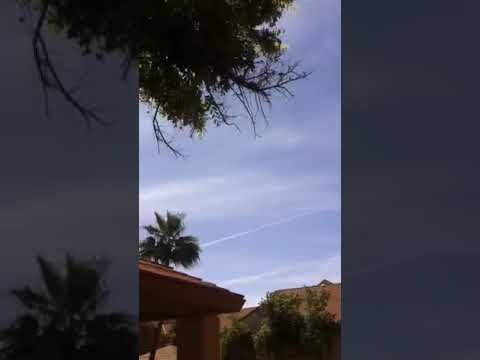In this blurry, low-quality vertical image, likely a screenshot from a video taken outdoors, the sky dominates the upper portion, displaying a deep blue backdrop with wispy clouds and white jet streams streaking across. Interspersed at the top are green leaves and branches, possibly from trees overhanging the scene. Towards the bottom of the image, there's a glimpse of a landscape featuring rocky or sandy hills, and on the bottom left, part of a clay-colored rooftop suggests the presence of a building. A prominent palm tree rises above this roof, adding a touch of lush green foliage. This outdoor setting, bathed in daylight without any visible sun, captures a mix of earthy browns, tans, and various shades of green against the expansive sky. The overall scene is serene and natural, devoid of any people or text.